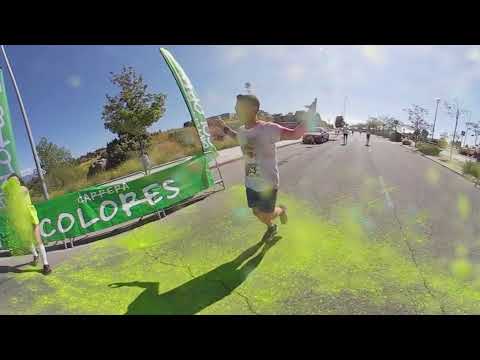A man with short, dark hair is jogging down a light gray asphalt street, one foot in the air behind him and his hands raised triumphantly. He is dressed in a white shirt, blue jean shorts, and black shoes. The ground beneath him is scattered with green paint, contributing to a festive atmosphere that suggests a race or celebratory event. To his left, a young girl in a light green outfit with white socks and dark shoes stands in front of a blotch of light green paint. Also to his left lies a green banner with white letters that read "Calpera Colores." Behind the banner rises a tree lush with green leaves, tilting slightly to the left. Further down the street, faint white lines guide a distant crowd of runners, and a red car is parked along the left curb. The sky is a clear blue with scattered white clouds, adding to the lively outdoor scene.